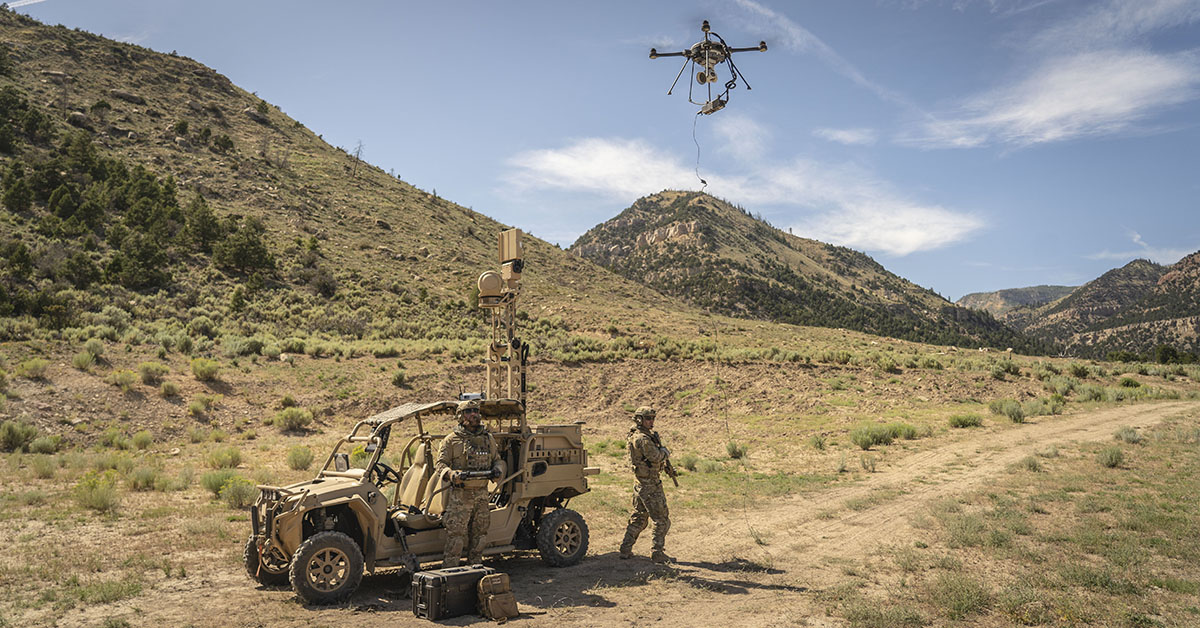In this detailed photograph of a military operation, two soldiers in full uniform are conducting a drone test in an arid, mountainous valley. The clear daytime skies and surrounding dry brush accentuate the rugged terrain. Parked on a dirt trail nearby is a small all-terrain military vehicle. One soldier, standing near the driver's side of the vehicle, is operating a remote control to fly a large drone, which is hovering approximately 15 feet above the ground. At his feet are a black utility case and a small backpack. The second soldier, armed with a large rifle pointed downward, stands on alert, scanning the surroundings for potential threats. The landscape is characterized by its tan and beige hues, interspersed with sparse patches of green vegetation. A well-worn path is visible, indicating the route they traveled.